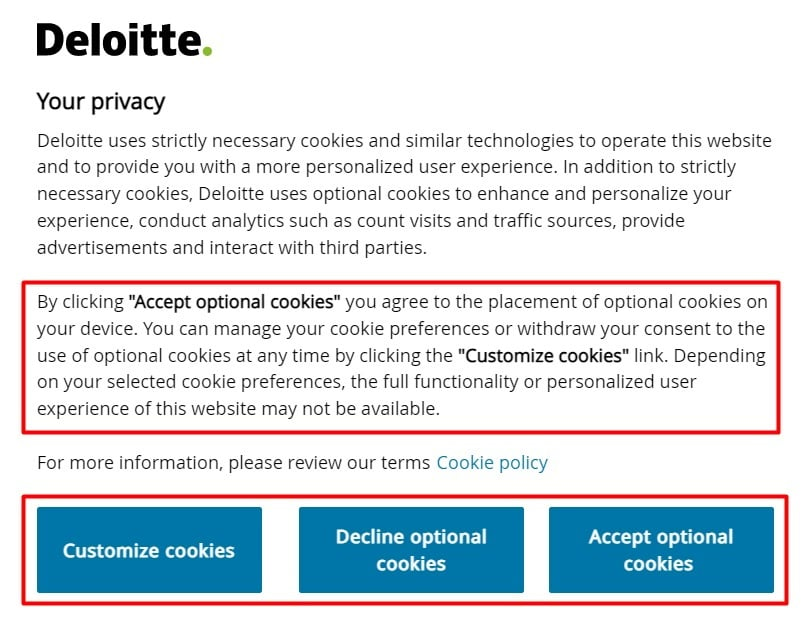The image represents a privacy policy web page for Deloitte, characterized by a predominantly white background, which blends seamlessly into the browser window, making the borders indistinguishable. 

At the top of the page, the Deloitte logo is prominently displayed in large, bold black letters, with a distinctive green period at the end. 

Beneath the logo, the heading "Your Privacy" appears in slightly smaller black text, emphasizing the focus of the page.

The body of the text, in a standard font slightly lighter and smaller than the "Your Privacy" heading, reads: "Deloitte uses Strictly Necessary Cookies and similar technologies to operate this website, and to provide you with a more personalized user experience. In addition to Strictly Necessary Cookies, Deloitte uses Optional Cookies to enhance and personalize your experience, conduct analytics such as count visits and traffic sources, provide advertisements, and interact with third parties."

Below this text, within a red-bordered box, is the following notice: "By clicking Accept Optional Cookies, you agree to the placement of Optional Cookies on your device. You can manage your cookie preferences or withdraw your consent for the use of Optional Cookies at any time by clicking Customize Cookies link. Depending on your selected cookie preferences, the full functionality or personalized user experience of this website may not be available. For more information, please review the terms and cookie policy."

Directly beneath this, still within the red-bordered box, are three blue buttons with white text inside them, labeled as "Customize Cookies," "Decline Optional Cookies," and "Accept Optional Cookies," providing users with options for managing their cookie preferences.